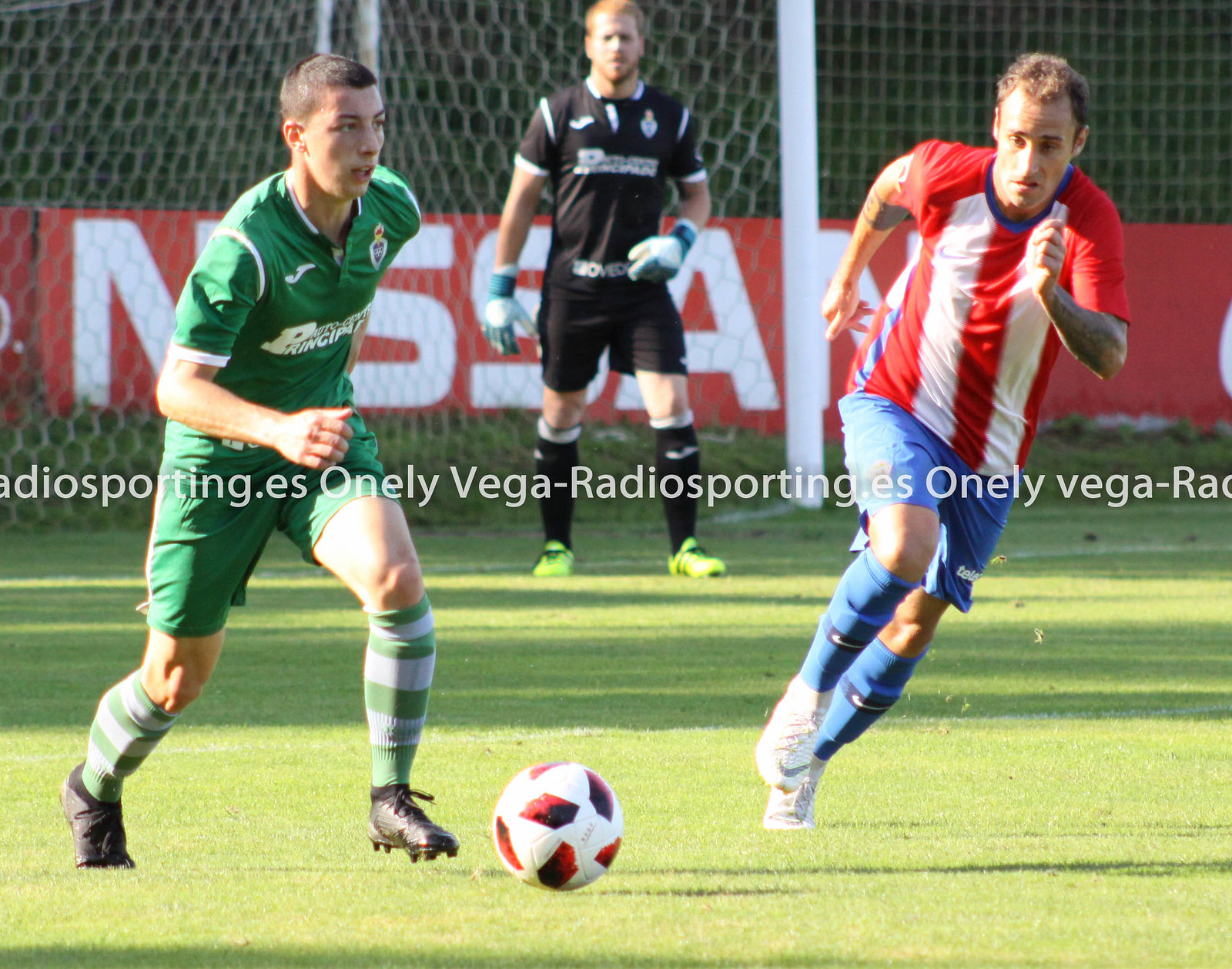In this vibrant outdoor photograph, three men are actively engaged in a soccer game on a well-maintained field. Dominating the background is a bright red rectangular sign emblazoned with the word "Nissan" in bold white letters, positioned behind a white netted soccer goal. Closest to this sign stands a man dressed in a black uniform with short red hair, adorned with white and green gloves and distinctive fluorescent green cleats, possibly indicating his role as the goalkeeper or an official.

At the forefront of the action are two soccer players converging towards a uniquely patterned soccer ball marked with red, white, and black boxes. The player on the left, sporting short buzzed brown hair, is captured mid-motion with his arm crooked as if running. He wears a striking green jersey complemented by green and white socks and black cleats. Opposite him, the player on the right, also with short brown hair, is visibly in stride with arms animated, dressed in a red and white striped jersey, blue shorts, blue socks, and white cleats. Both players, appearing to be white males, are intensely focused on the dynamic play unfolding before them.